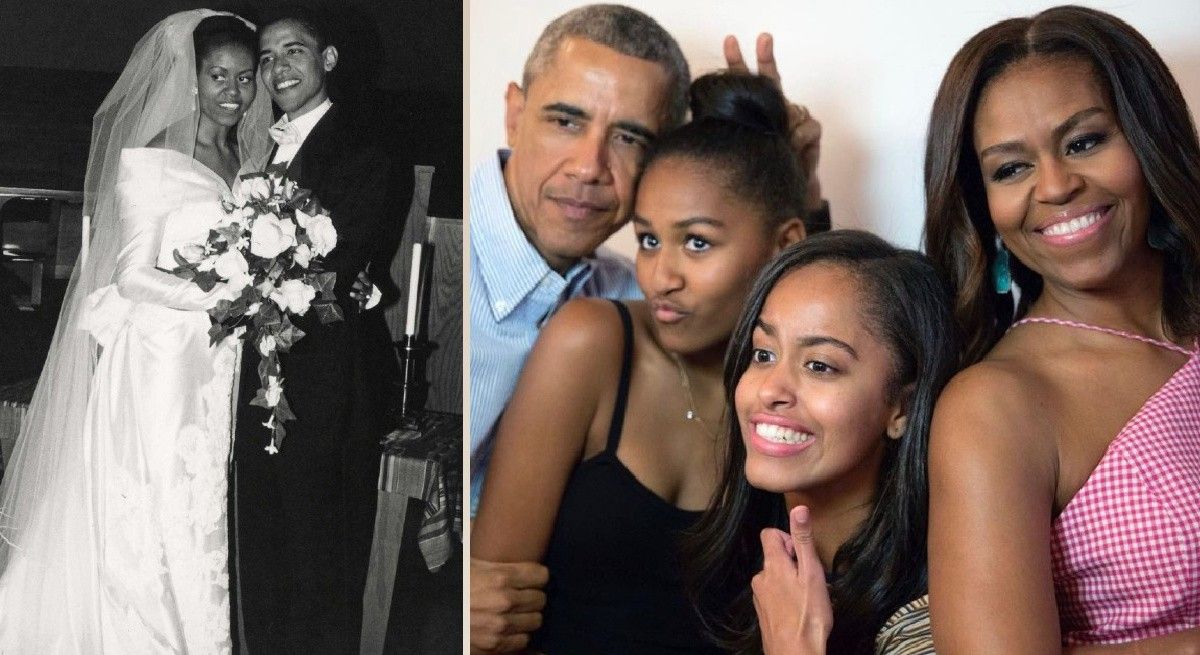The image consists of two photographs juxtaposed. On the left, there's a black-and-white wedding photograph of Michelle and Barack Obama. Michelle is adorned in an elegant over-the-shoulder, long-sleeved white wedding gown with a large, long veil, and she holds a substantial bouquet of roses. Beside her, Barack is elegantly dressed in a black tuxedo. They are embracing and smiling warmly at the camera, with a candlestick visible on a nearby table, suggesting the intimate setting of the church.

On the right, there's a more recent color photograph of the Obama family. Barack, now wearing a blue button-up shirt, stands to the left making a playful bunny-ear gesture behind one of his daughters. The daughter with her hair in a bun, wearing a black spaghetti strap top with a necklace, stands next to him. Beside her is her sister, with her hair down and making a silly face. On the far right stands Michelle Obama, dressed in a gingham checkered off-the-shoulder tank top, smiling. The entire family exudes a sense of joy and togetherness, with each member displaying their unique personas through their expressions and gestures.